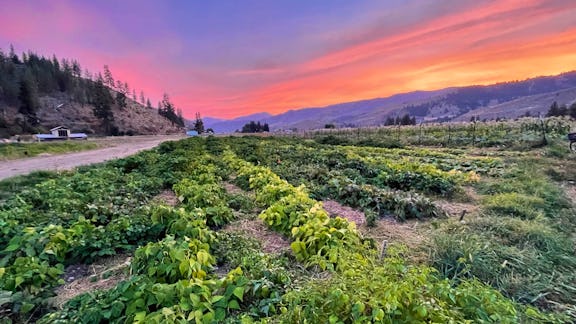The image captures a serene and colorful countryside at sunset. In the foreground, lush rows of crops are planted meticulously, with narrow paths for tending the plants. The crops include low-lying vegetables and possibly taller stalks like corn. A dirt road runs along the left side of the field, leading into the background. There, a barn-like structure, perhaps a barn, can be discerned. In the distance, towering mountains frame the horizon, crowned by a vibrant sky awash with hues of orange, yellow, pink, purple, and red. The scene also includes a small hill topped with several trees to the left of the field, and there appears to be a hint of a blue structure, possibly a house, further down the road. The photograph is a breathtaking depiction of rural tranquility.